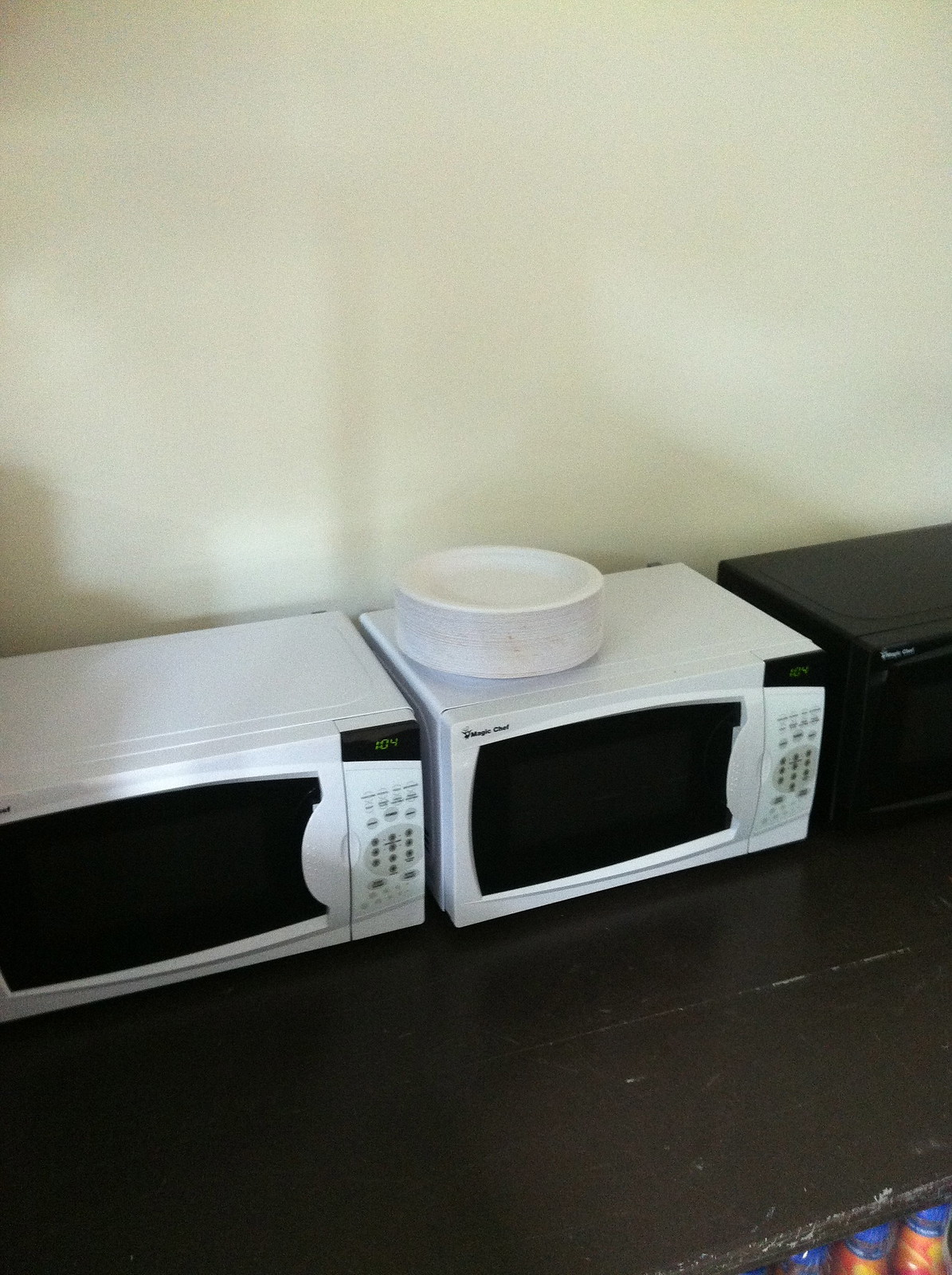In this indoor photograph, we see a close-up of a dark brown or black table with a few scuff marks on the edge and three microwaves positioned side by side on top of it. The leftmost and middle microwaves are white and appear nearly identical, both displaying the time 1:04 in the upper right-hand corner of their black screens. Each of these microwaves has a button panel on the right side. The middle microwave has a stack of white paper plates placed on top of it. The third microwave on the right is black and partially visible due to being cut off in the image, making it difficult to discern details such as the door or button features. However, it shares the same company logo at the top left corner, albeit slightly off-center, as the middle microwave. Beneath the table, several bottles with orange and blue caps are partially visible in the bottom right corner. The background features a smooth, cream-colored wall with some shadowing behind the microwaves.